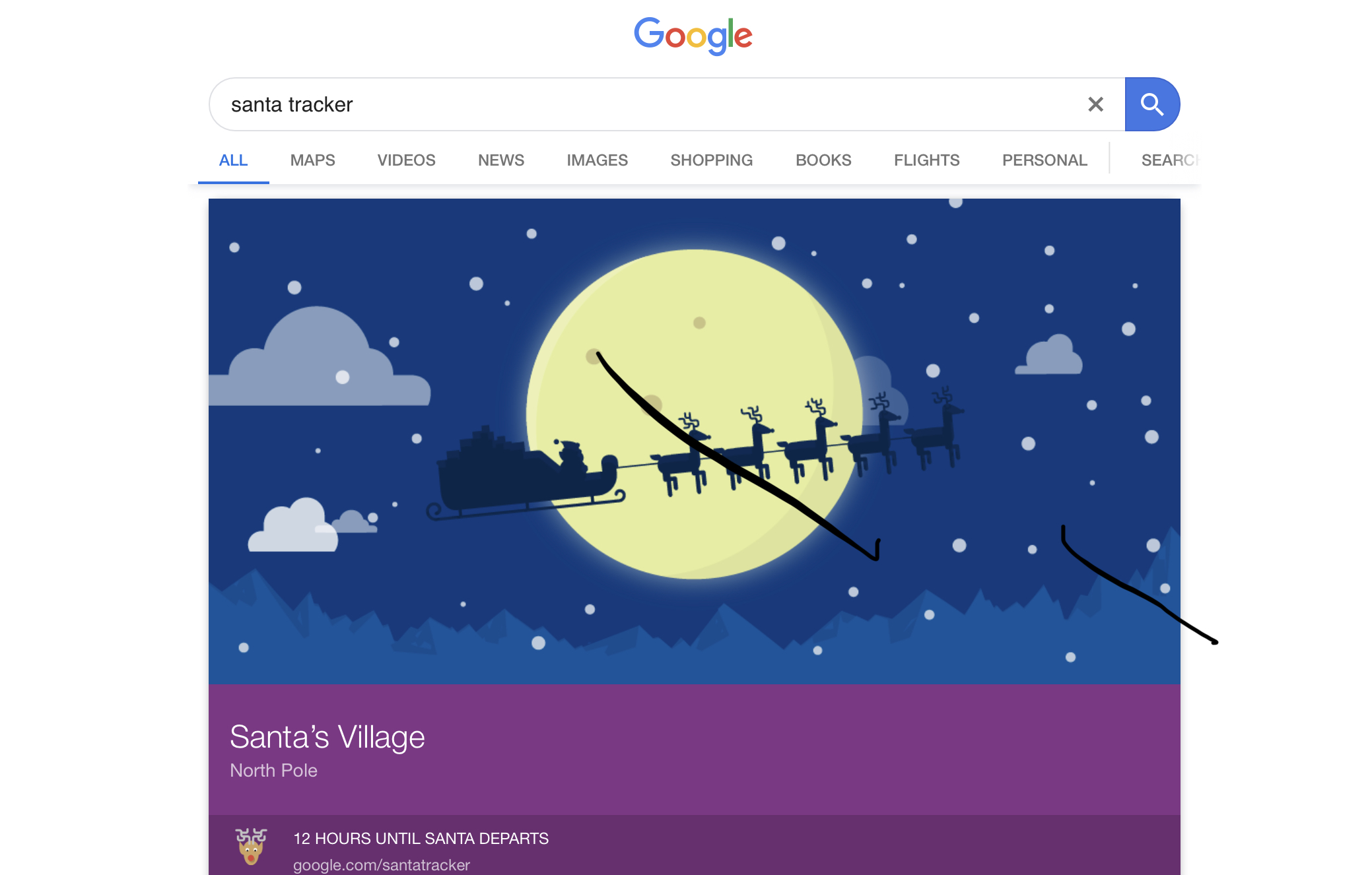The image appears to depict a Santa Tracker webpage with a festive design. At the top center, the "Google" logo is prominently displayed, with capitalized, multi-colored letters: the 'G' is blue, the first 'O' is red, the second 'O' is yellow, the lowercase 'g' is blue, the 'l' is green, and the 'e' is red. Below the logo, a search bar is featured with "Santa Tracker" typed into it. To its right, there is an 'X' icon followed by a blue search button with white text.

Underneath the search bar, several headers are listed: "All," "Maps," "Videos," "News," "Images," "Shopping," "Books," "Flights," "Personal," each in black text, except for "All," which is highlighted in blue.

The main image shows Santa Claus in a sleigh being pulled by five reindeer, silhouetted against a dark blue sky. A large pale yellow moon, stars, and clouds add to the night sky's ambiance. Below this scene, a light blue mountain range is visible.

At the bottom of the image, a purple bar with white text reads "Santa’s Village North Pole." Below this, a darker purple bar features a small reindeer icon on the lower left and text stating, "12 hours until Santa departs." A URL, "google.com/santatracker," is displayed below this announcement.